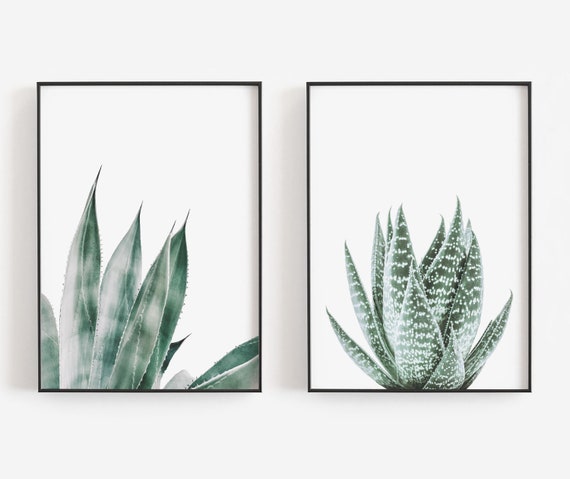The image displays two framed portraits of what appear to be aloe vera plants, set side-by-side on a white wall. Both portraits are encased in thin black frames and feature a pure white backdrop, accentuating the central focus on the plants. The left portrait offers a close-up view of aloe vera leaves that are green with lighter shades in some areas. These leaves end in a sharp tip and display subtle spikes. The right portrait showcases the entire body of the plant, with its leaves rising upward in a pattern reminiscent of an artichoke. These leaves are also green but distinguished by a multitude of white spots and speckles. Each portrait captures the intricate details and textures of the aloe vera plants, highlighting their unique patterns and forms.